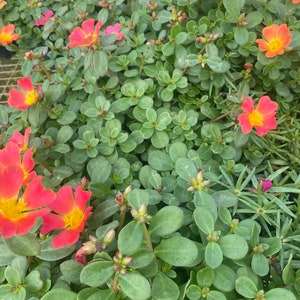This image is a detailed close-up of a vibrant, outdoor plant grouping taken from above, displaying a vivid mixture of greenery and vibrant flowers. Dominating the composition are the rich, green oval-shaped leaves, each marked by a distinct central vein. Toward the bottom right, a cluster of spiky leaves adds texture to the scene. Interspersed among the greenery, succulent plants with thick, rounded leaves suggest a water-retaining characteristic, hinting at their resilience.

The standout feature of the image is the array of hot pink flowers with striking yellow circular centers. These flowers appear throughout the image, with several positioned in the bottom left corner and along the image's edges, creating a harmonious border. A noteworthy detail is one flower bud, dark pink in color, waiting to bloom. Together, the diverse plant textures and the vivid hues of the flowers transform the scene into a dynamic, almost painterly depiction of nature's beauty, possibly indicative of a carefully cultivated nursery or vibrant garden bed.